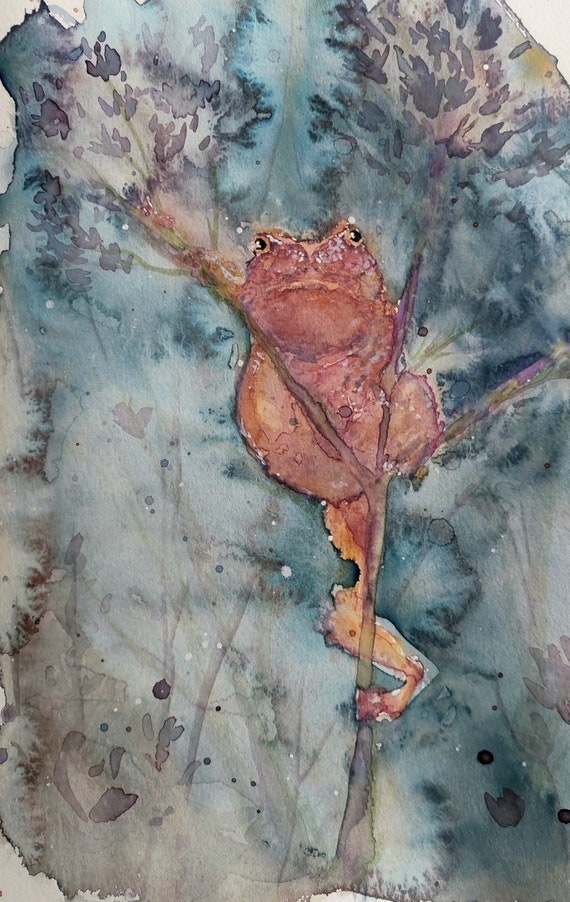This is a detailed watercolor painting featuring a toad as its focal point. Set against a rich, natural backdrop dominated by shades of green and brown, with a bluish-green hue reminiscent of a dense forest scene, the painting captures a tranquil outdoor environment. In the foreground, a small, branching stem forks into three sections, providing a perch for the toad. The toad, colored in a burnt-orange or brownish-pink shade, appears to be climbing the stem, its legs positioned as though mid-movement. The background, though primarily green and brown, also contains subtle hints of blue, gray, and purple, enhancing the mystic, forest-like ambiance of the scene. The edges of the painting remain uncolored, revealing the white paper or canvas it was created on, emphasizing the central image and reinforcing the watercolor aesthetic.